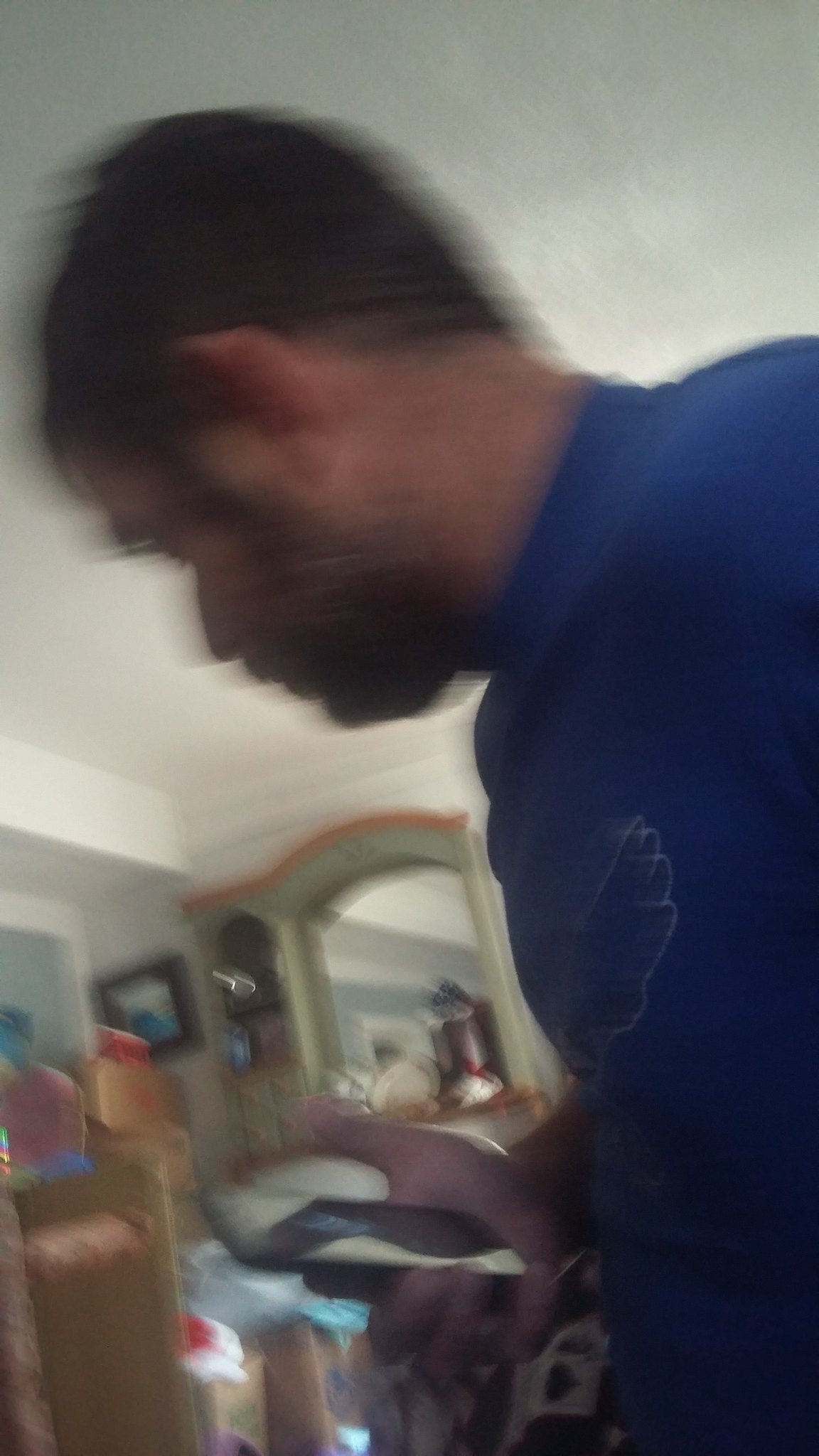In this image, a slightly blurry close-up captures a man in profile. He has neatly trimmed, very short dark hair, and sports a beard and mustache. Dressed in a royal blue crewneck shirt adorned with a white design on the front, he stands inside a home environment, concentrating intently on his cell phone held in his right hand. Just in front of him is a cluttered countertop, featuring a tall brown box and various bags. In the background, a mantle embellished with a mirror and framing an arched piece above a fireplace adds to the cozy ambiance of the scene. The man appears absorbed in reading something on his screen amidst a day at home.